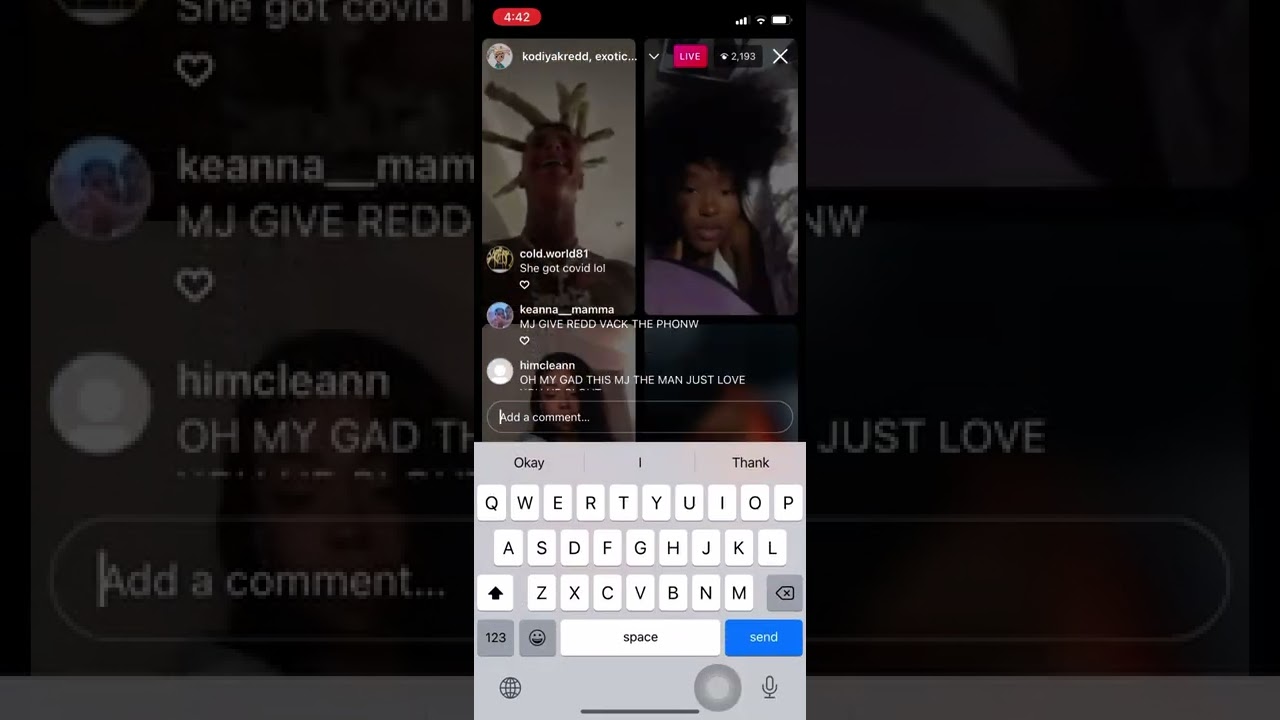This screenshot captures a horizontally oriented image with a grayish background. Although it is slightly shorter than a typical landscape image, its dimensions appear to be approximately 35:65, providing a general idea of the proportions and orientation.

In the background, the scene depicts comments on a video. At the top of the comments, one reads, "she got COVID." Below that, user Kiana_M_A_M has posted "MJ give REDD," and underneath, HimClean with two N's comments, "oh my god, something just love."

Superimposed over this background, there's a screenshot of a mobile phone. The phone display shows a selection of videos. On the left, there’s a video of a man with long, pale green dreadlocks. To the right, there is a Black woman with an afro. In the bottom left, there appears to be a video of singer Billie Eilish. The video in the bottom right corner is too blurred to identify.

Additionally, the phone's screen reveals suggested text options, which are "OK," "I," and "thank."